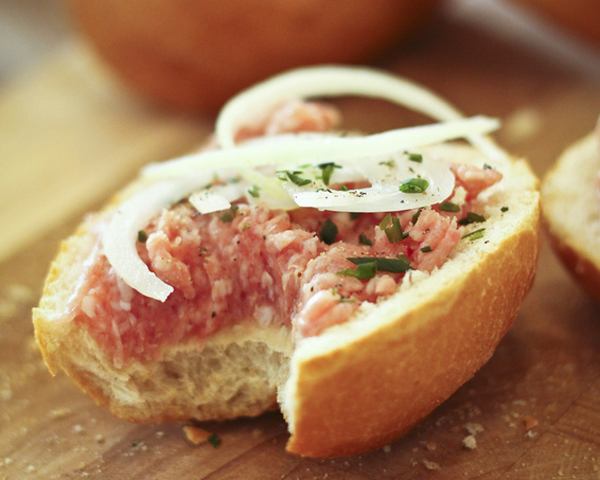The image displays a traditional German Mettbrötchen, featuring a crusty brown roll halved and generously layered with seasoned raw minced pork, known as "Mett." The finely ground pink meat, which may appear uncooked to the unfamiliar eye, is indeed prepared for consumption in this manner. Atop the Mett are several rings of fresh white onion, with three prominent thicker slices visible. The combination is garnished with a sprinkling of chopped chives and a delicate dusting of seasoning, enhancing its visual and aromatic appeal. In the background, part of the upper half of the roll is partially visible, resting on a rustic brown wooden table or butcher block. The setting is further detailed with a vague appearance of a round, grapefruit-like object, adding a touch of curiosity to the scene.